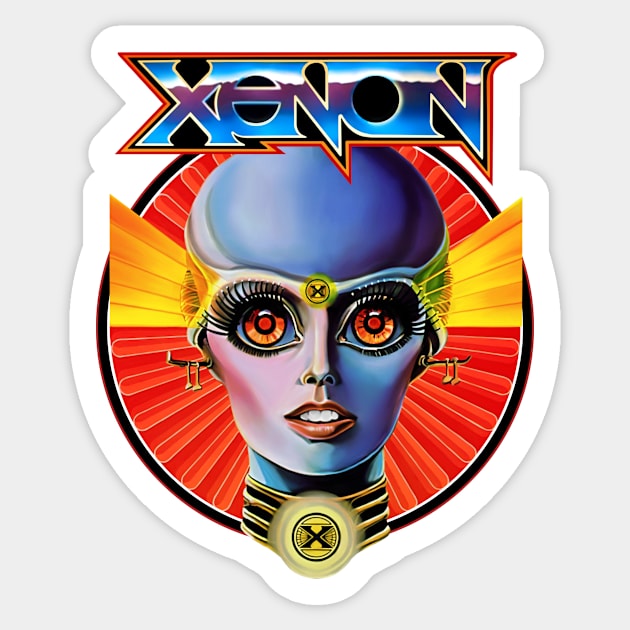The image depicts a striking piece of artwork, possibly a digital illustration or a conceptual mock-up of a sticker or patch, set against a solid gray background. Dominating the upper section of the artwork, the word "Xenon" is prominently displayed in white, blue, and purple block letters with a red outline. Beneath this title is the compelling image of a futuristic or alien female figure.

She has a bald, blue-skinned head with varied shades of purple accentuating her features. Her enormous, orange-red eyes are double the size of human eyes and are framed by long, black eyelashes above her open mouth with red lips and white teeth. A small, golden button or decorative element is positioned between her eyes.

The figure wears a gold and black choker around her neck that features a prominent black "X" at the front, resembling a piece of armor or the base of a light bulb. The same "X" can also be found on her forehead, adding to her mysterious allure. Golden earrings that protrude from her ears add to her striking appearance.

She is surrounded by rays of light in shades of red, orange, and yellow, all outlined in black. This vibrant radiance is further enclosed within an off-gray square that stands out against the larger solid gray background. The entire composition is framed by a white border, creating a vivid, otherworldly portrait that captivates the viewer's attention.